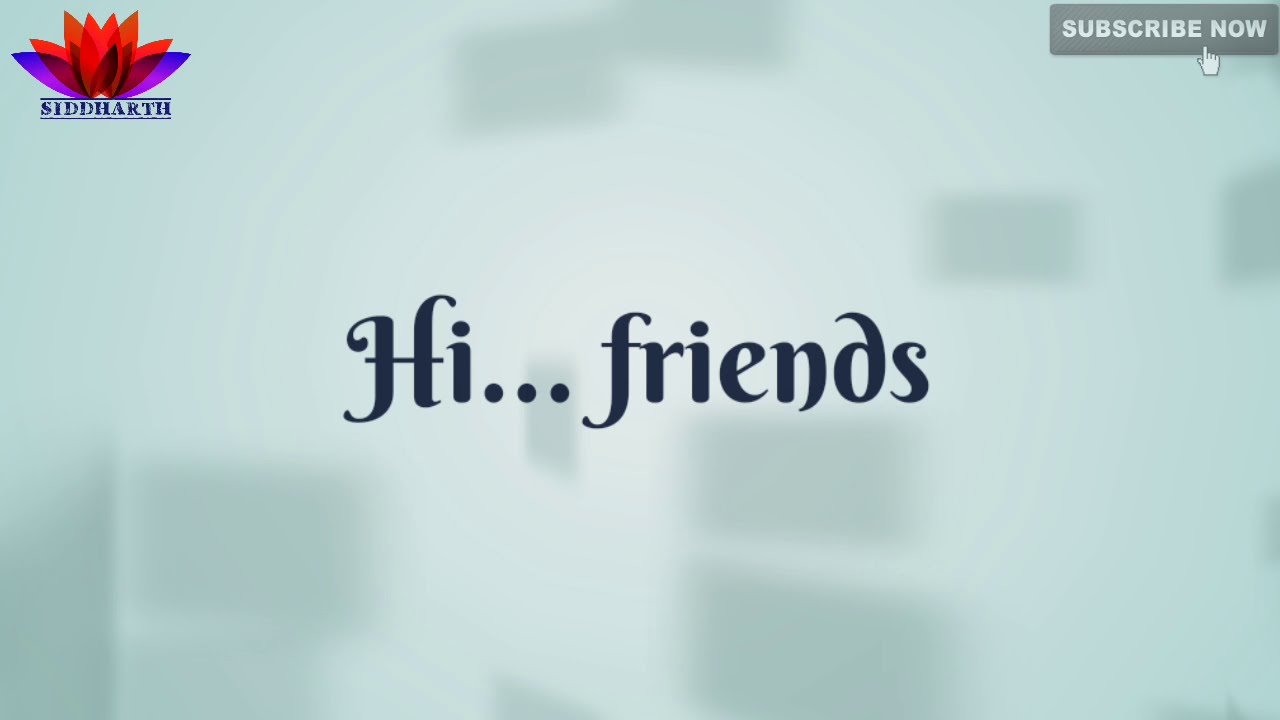The image appears to be a screenshot, likely from a YouTube video or a similar streaming platform, with a predominantly light gray to greenish-gray background punctuated by medium to dark gray blurry rectangles. In the upper right corner, there's a horizontal gray rectangle with white text reading "SUBSCRIBE NOW," alongside a mouse pointer graphic. On the upper left, there's a flowery logo with petals ranging from purple to red, and beneath it, in blue text, is the name "Siddharth" with a horizontal purple line above and below the name. Centered in the middle of the image, there is dark blue to black stylized text saying "Hi... friends," with a looping and curved font style. The overall composition suggests a designed splash screen intended to prompt viewers to subscribe.